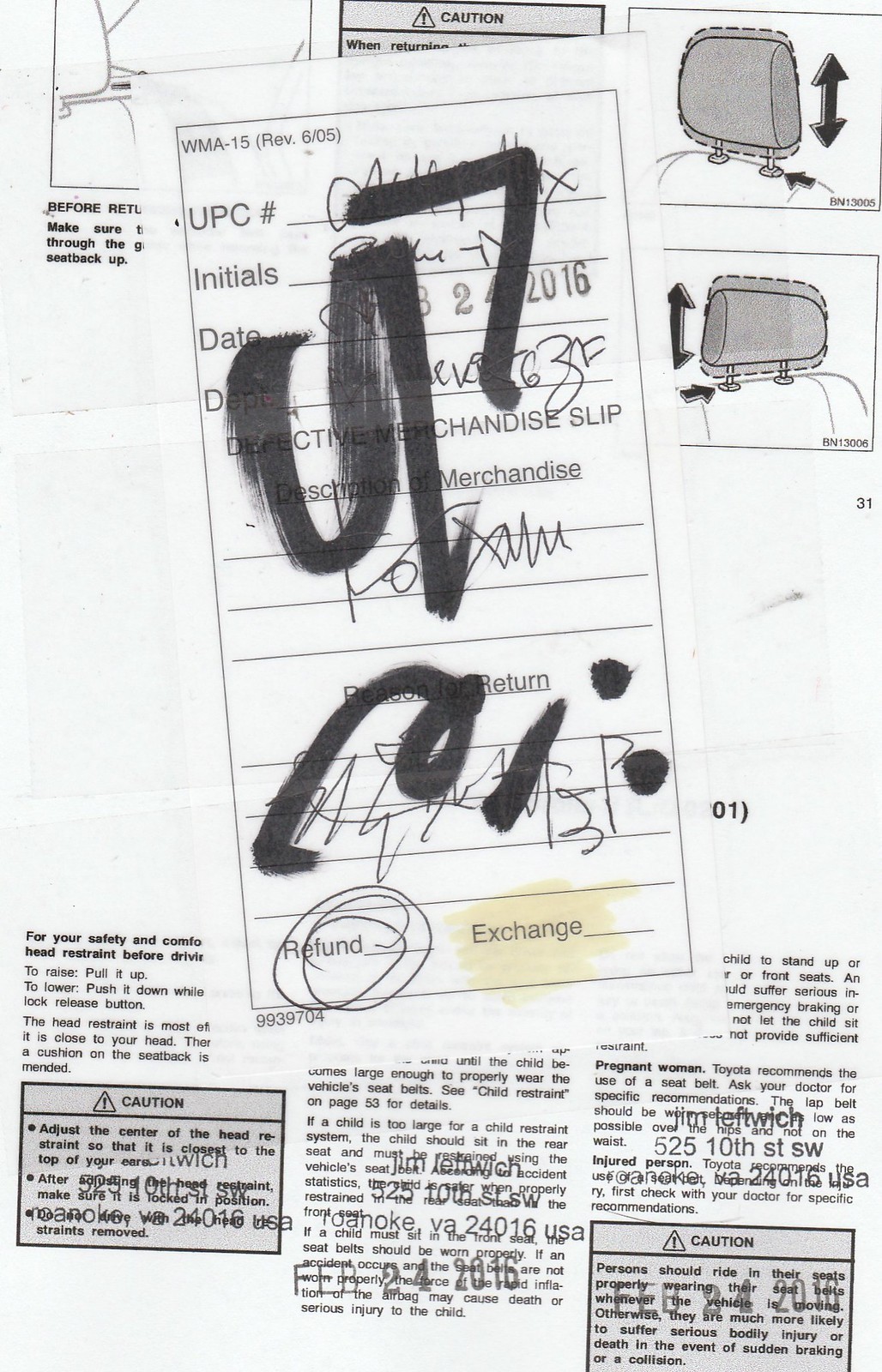The image depicts a user manual page related to a car headrest, overlaid with a defective merchandise slip. The slip is predominantly white with black text and includes various details such as a UPC number, initials, and a date from 2016. The slip clearly indicates it is for defective merchandise, highlighted by a prominent "refund" note circled and accompanied by a signature. The manual page underneath features a black and white image of a car seat with a headrest, including arrows pointing to specific parts. The accompanying text on the manual page is somewhat blurry and in black font, making it hard to read.